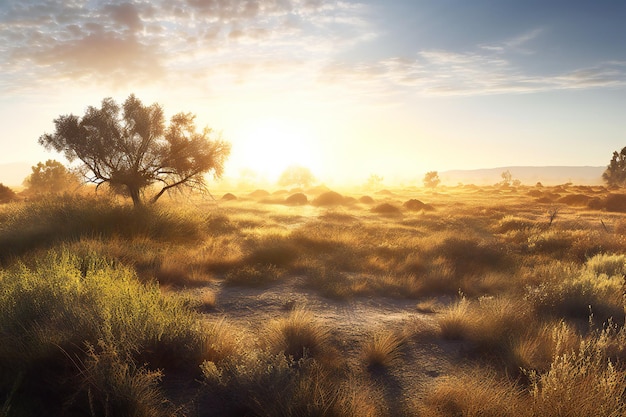The image depicts a serene, almost dream-like landscape that could be located in Africa, Australia, or even the prairie lands of America. The landscape features a mixture of golden, tall grasses growing in clumps and patches of sandy ground that extend far into the distance. Scattered across the scene are small trees with bare trunks and leafy canopies, adding to the sparse, yet captivating, environment. The sun, positioned low in the sky, illuminates the entire scene with a golden hue, creating a subtle haze that diffuses the light, giving the grasses a fluid, almost water-like quality. The sky is a soft blue with a few gray and white clouds, contributing to the peaceful and somewhat lonely atmosphere, devoid of any animals, birds, or humans. The palette of colors in the image includes greens, yellows, whites, blues, browns, and beiges, further enriching the natural beauty of this vast, tranquil landscape.